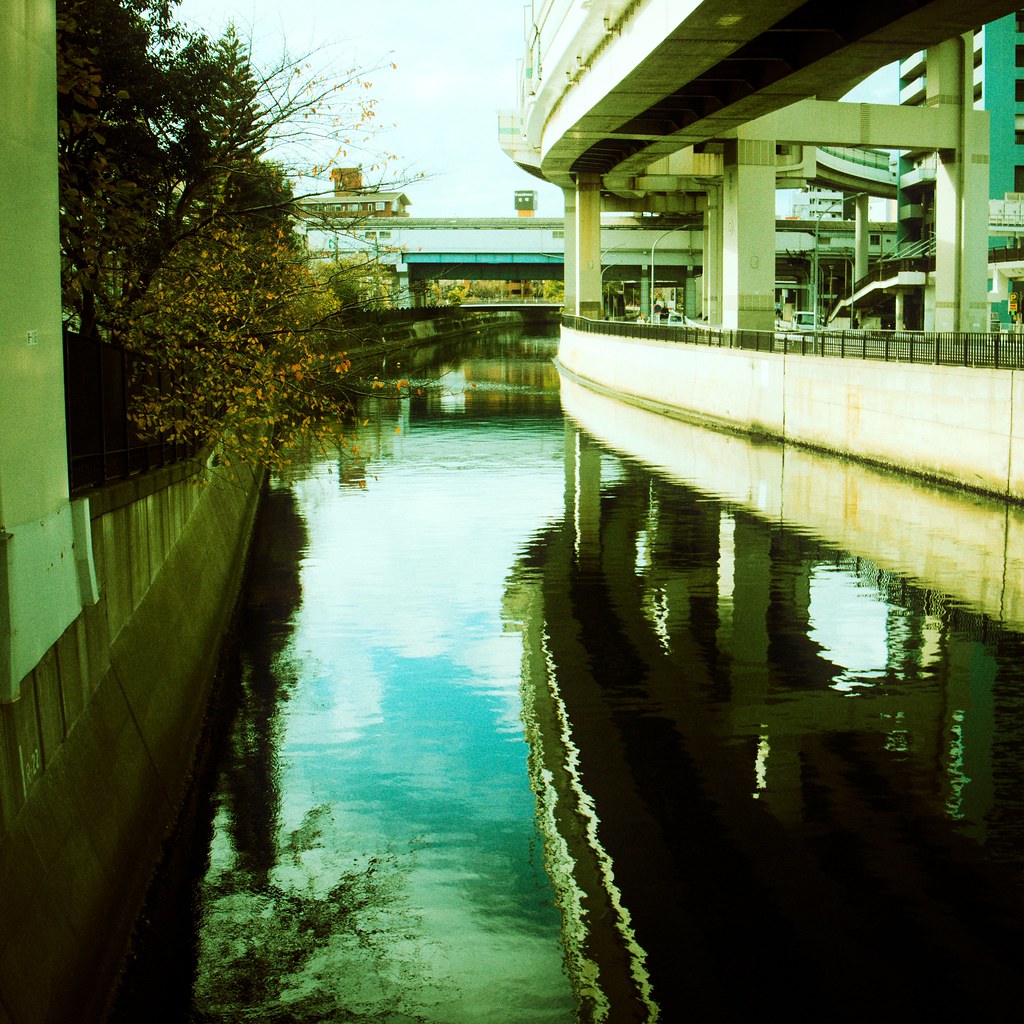This photograph captures an urban scene featuring a waterway, most likely a man-made canal or reservoir, bordered by various structures. Prominently reflected in the calm water is a two-story elevated railway or roadway, supported by I-beams and metal structures. This structure, curving off to the right, seems to lead into the city, where a train station-like building can be observed in the background. On the left side of the photo, a brown tree with dying leaves, indicative of autumn, overhangs a large concrete wall that runs alongside the canal. An adjacent stairwell ascends to a green complex building positioned near the bottom right of the scene. Additional elements include green road signs with white writing, typical of freeway signage, and a cement wall featuring a gate pipe, adding to the urban infrastructure surrounding the waterway.